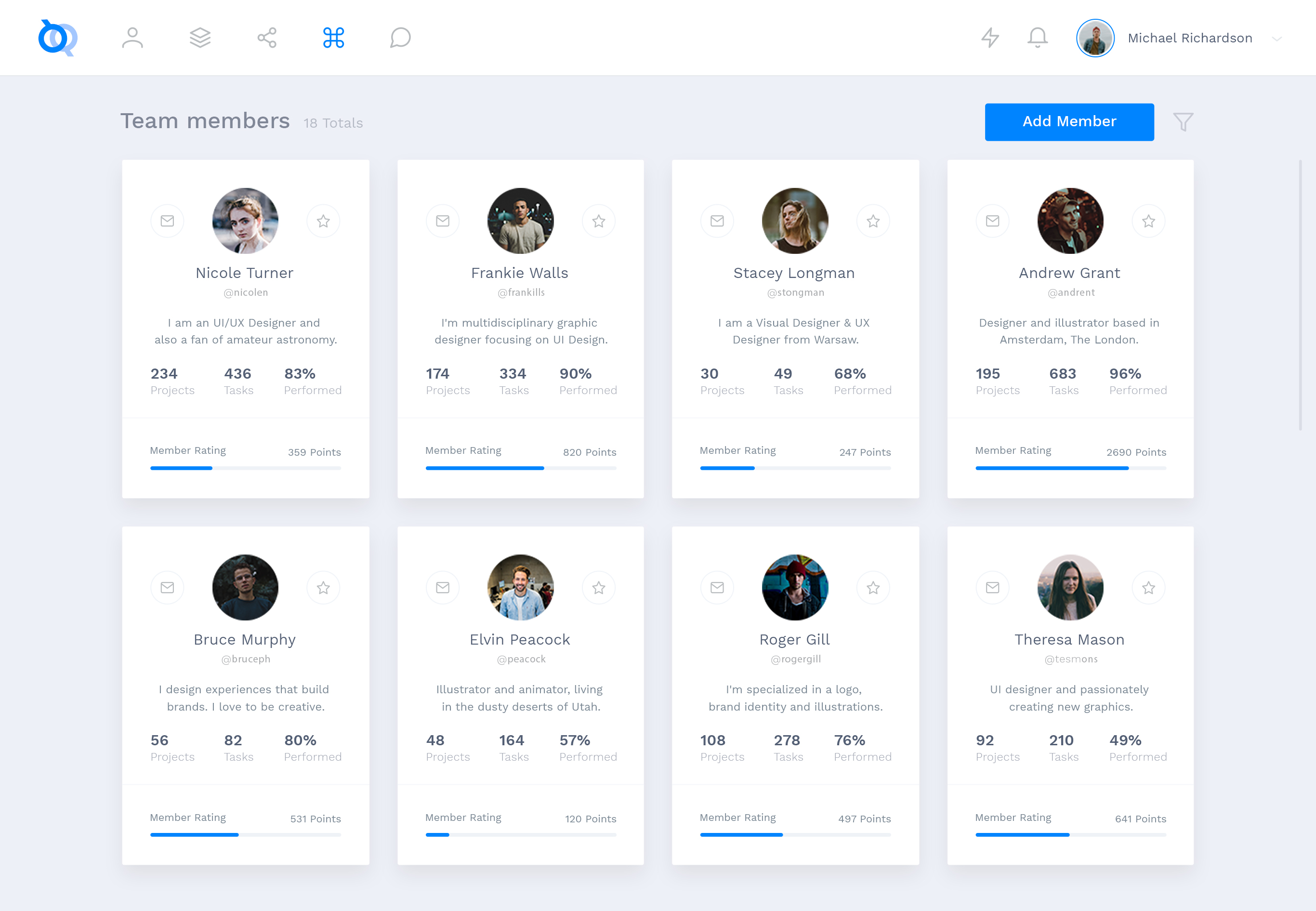This image, captured on a personal device, displays a profile view of team members using a management or collaboration application. The screen shows an overview indicating a total of 18 team members, though it currently only displays 8, organized in two rows of four.

In the top row, starting from the left:
1. **Nicole**: Identified as a UI/UX Designer with a passion for amateur astronomy. She has completed 234 projects and 436 tasks, boasting an 83% performance rate. Nicole's member rating is 359 points, visually represented by a progress bar filled approximately one-third of the way with blue.
2. **Frankie Walls**: A multidisciplinary graphic designer emphasizing UI design. Frankie's performance is marked by a significantly longer progress bar, indicating an impressive 820 points.
3. **Stacey Logman**: A visual and UX designer from Warsaw. She holds 247 points on her member rating.
4. **Andrew Grant**: A designer and illustrator operating between Amsterdam and London. Andrew boasts a high member rating with 2,690 points.

In the bottom row, extending left to right, the remaining four team members are hinted at, though their details are not elaborated in this description.

This detailed caption reflects the structured layout and individual achievements of the visible team members, showcasing a snapshot of their contributions and expertise within the team.